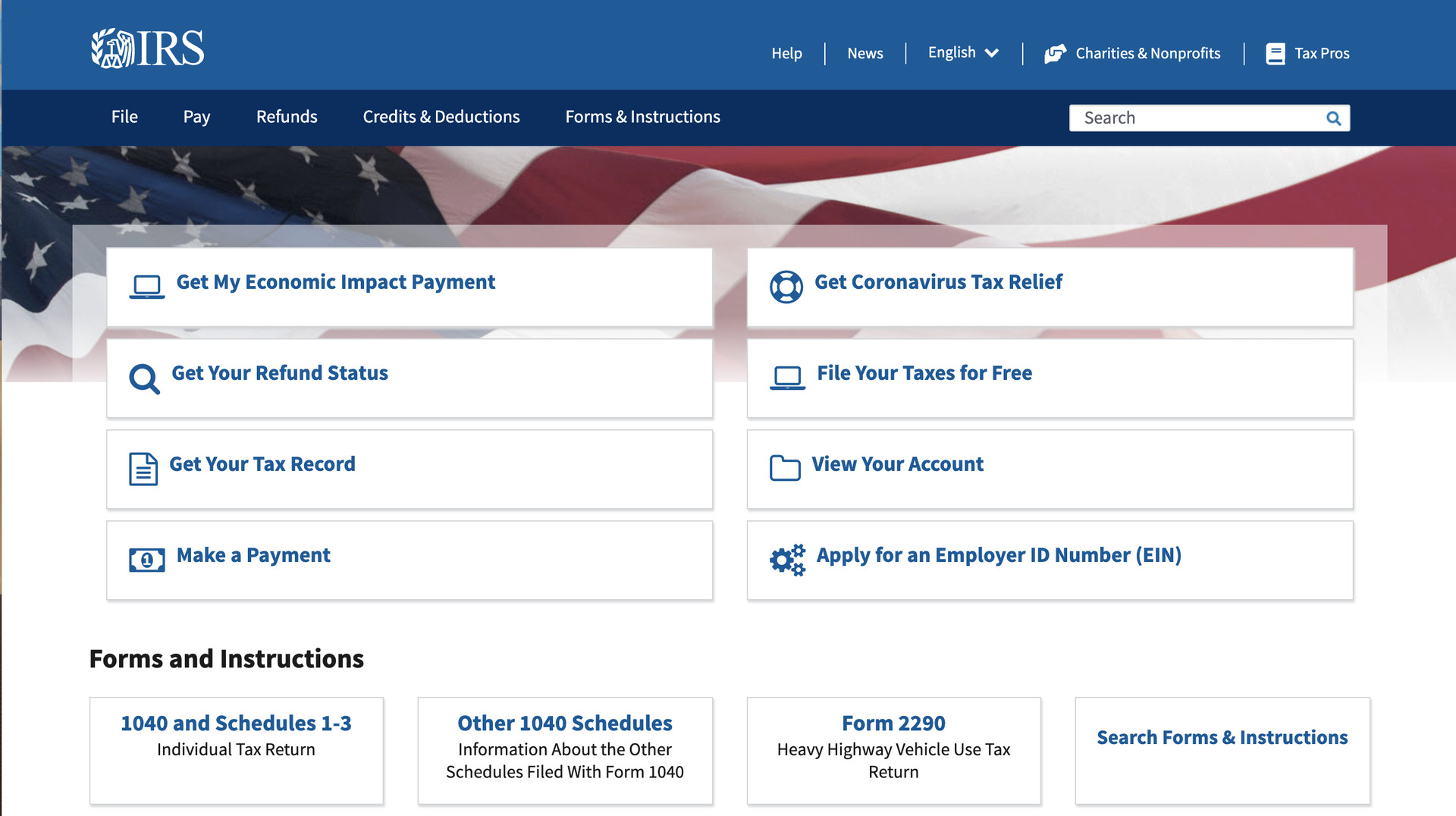Detailed Caption: A screenshot of the IRS website. The top section features two horizontal blue bars; the upper one is a lighter shade and the lower one a darker shade. The lighter blue bar displays the IRS logo, which seems to incorporate laurel leaves and possibly an eagle. Adjacent to the logo, the bar includes links labeled "Help," "News," "English," "Charities and Nonprofits," and "Tax Pros." Next to the "Charities and Nonprofits" link, there is an icon resembling a piece of paper with an arrow, and beside "Tax Pros," there's an icon that looks like an outlined document with textual markings.

Beneath this, the darker blue bar contains links labeled "File," "Pay," "Refunds," "Credits & Deductions," and "Forms & Instructions." 

Further down, there is a banner that incorporates elements of the American flag with red, white, and blue colors, along with stars. Below this banner, several rectangular white boxes with blue text are distributed across the screen. On one side, these boxes are captioned with:
- "Get My Economic Impact Payment" (accompanied by a laptop icon)
- "Get Your Refund Status" (with a magnifying glass icon)
- "Get Your Tax Record" (featuring a document icon)
- "Make a Payment" (alongside a dollar bill icon)

On the opposite side, another set of items includes:
- "Get Coronavirus Tax Relief" (with a circular logo)
- "File Your Taxes for Free" (paired with a laptop icon)
- "View Your Account" (with cogwheels icon)
- "Apply for an Employer ID Number (EIN)" (illustrated with a manila folder icon)

The bottom portion of the screen features a section with more options in black font reading "Forms & Instructions." This area contains four more white boxes with blue and black text that detail:
- "1040 and Schedules 1-3 Individual Tax Return"
- "Other 1040 Schedules: Information about the other schedules filed with Form 1040"
- "Form 2290: Heavy Highway Vehicle Use Tax Return"
- A search field labeled "Search Forms and Instructions"